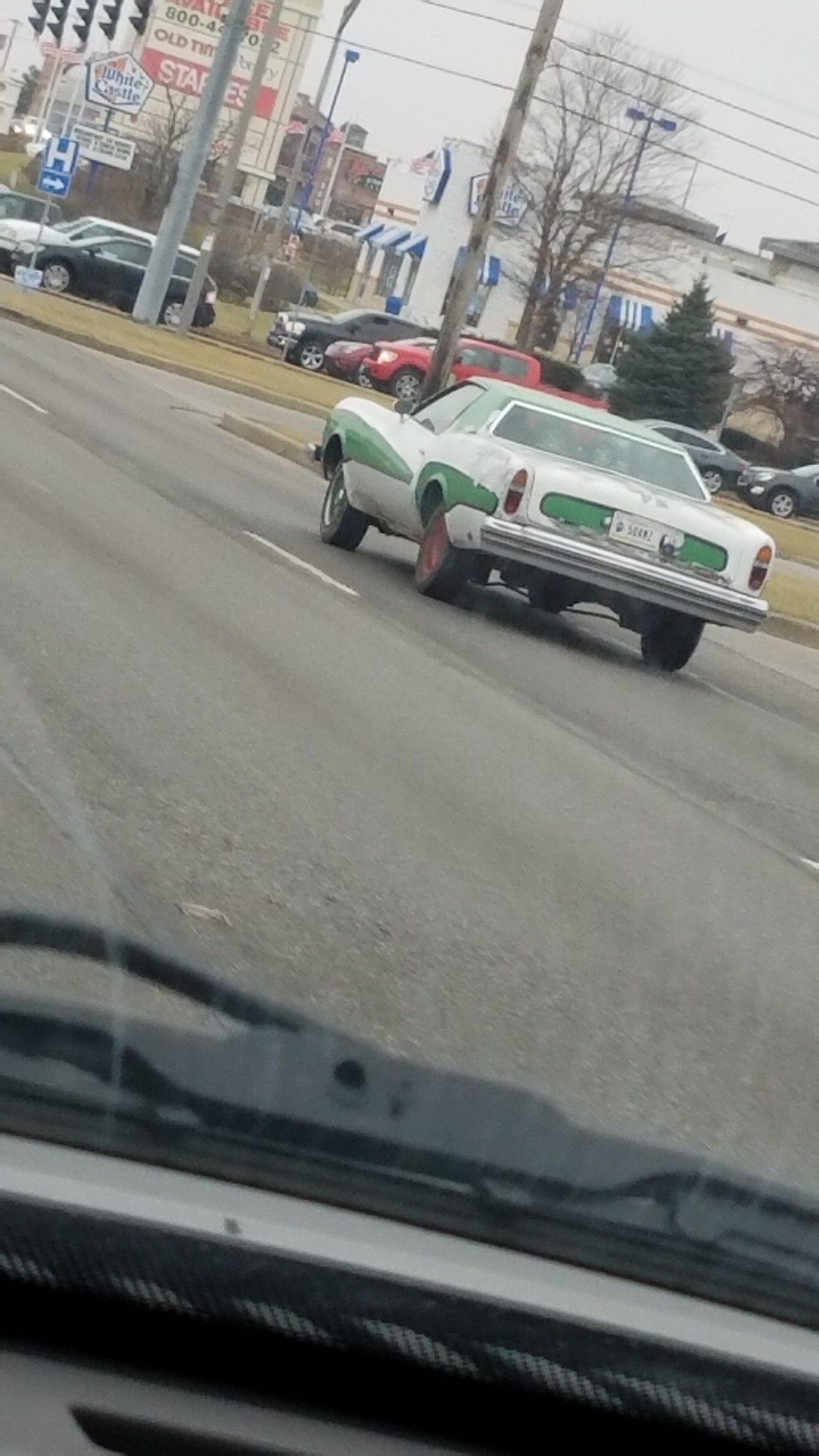The image captures a driver's-eye view of a city street through a car's windshield, complete with visible black windshield wipers at the bottom of the frame. Directly ahead on the road is a distinctive white and green muscle car convertible, identifiable by its gray vinyl roof and a missing hubcap on the driver's side rear wheel. The muscle car's green detailing is apparent along the sides and around the trunk area, near the license plate. To the right side of the image is a fast food building, likely a White Castle, which features blue awnings with white stripes. The road itself is marked by periodic white dashes and leads to an intersection where several vehicles, including a black car, a red pickup truck, a black pickup truck, and a few gray cars, are stopped at a red light. In the background, there is a strip mall sign for Staples, a telephone pole, and clear skies occupying the top right corner of the image.